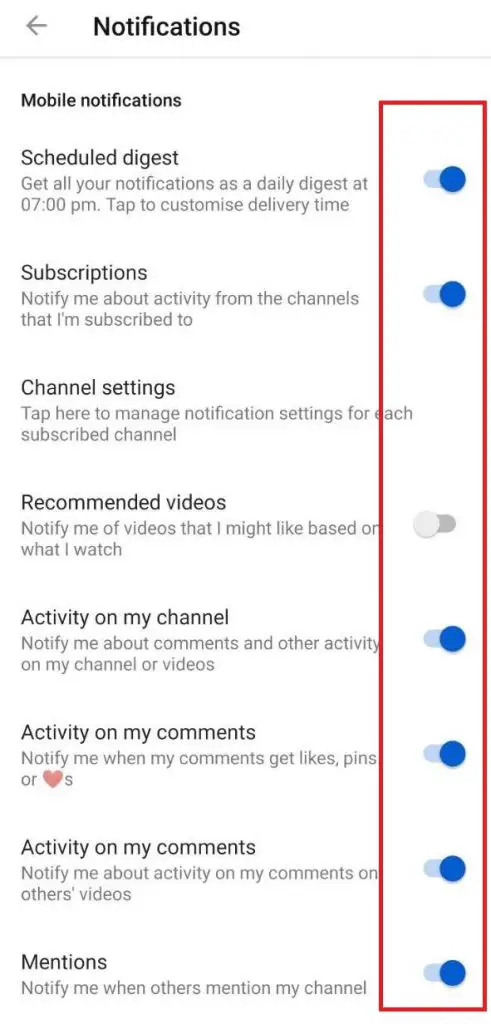This screenshot displays a section of a mobile notification settings page, characterized by a white background with black text. At the top, a gray back arrow is followed by the title "Notifications" in bold black lettering. Below this, a thin gray line separates the title from the first sub-section titled "Mobile Notifications."

The content is organized into various notification categories, each accompanied by a brief description and an adjustable setting, represented by a blue or gray circle. The active settings feature a blue circle icon, indicating they are turned on, while inactive ones have a gray circle.

1. **Scheduled Digest:** "Get all your notifications as a daily digest at 7 p.m. Tap to customize delivery time." This setting is active, indicated by the blue circle.
   
2. **Subscriptions:** "Notify me about activity from the channels that I'm subscribed to." This setting is active, shown by the blue circle.

3. **Channel Settings:** "Tap here to manage notification settings for each subscribed channel." This option is highlighted but does not feature a circle icon like the other settings.

4. **Recommended Videos:** "Notify me of videos that I might like based on what I watch." This is the only inactive setting, noted by the gray circle.

5. **Activity on My Channel:** "Notify me about comments and other activity on my channel or videos." This setting is active, with a blue circle.

6. **Activity on My Comments:** "Notify me when my comments get likes, pins." This setting is active and indicated by a blue circle, with a red heart icon and the letter 'S' next to it.

7. **Activity on My Comments on Others' Videos:** "Notify me about activity in my comments on others' videos." It is also an active setting, displayed by a blue circle.

8. **Mentions:** "Notify me when others mention my channel." This setting is active, shown by the blue circle.

All the settings, except for "Channel Settings," are encapsulated within a long red box that emphasizes the section comprising these options.